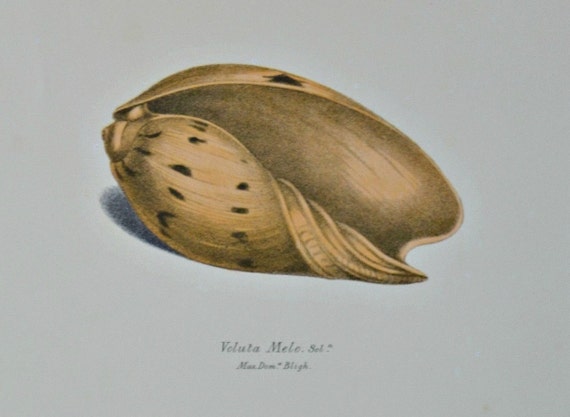This image depicts an artist's rendering of a seashell resting on a medium gray background. The shell, which resembles a cracked-open nut or perhaps an acorn, has a light to dark brown exterior with scattered black spots primarily on the top and left side. The shell is opened, revealing a darker brown interior that can be seen through the curled, grooved lower right section. Its surface showcases folds and a smooth top with the largest dark patch. The shell is light brown on the outside and is egg-shaped, lying horizontally with its shadow cast to the left. Below the shell, there is small black text that appears to read "Bilater Milo SD", although some letters may be unclear.